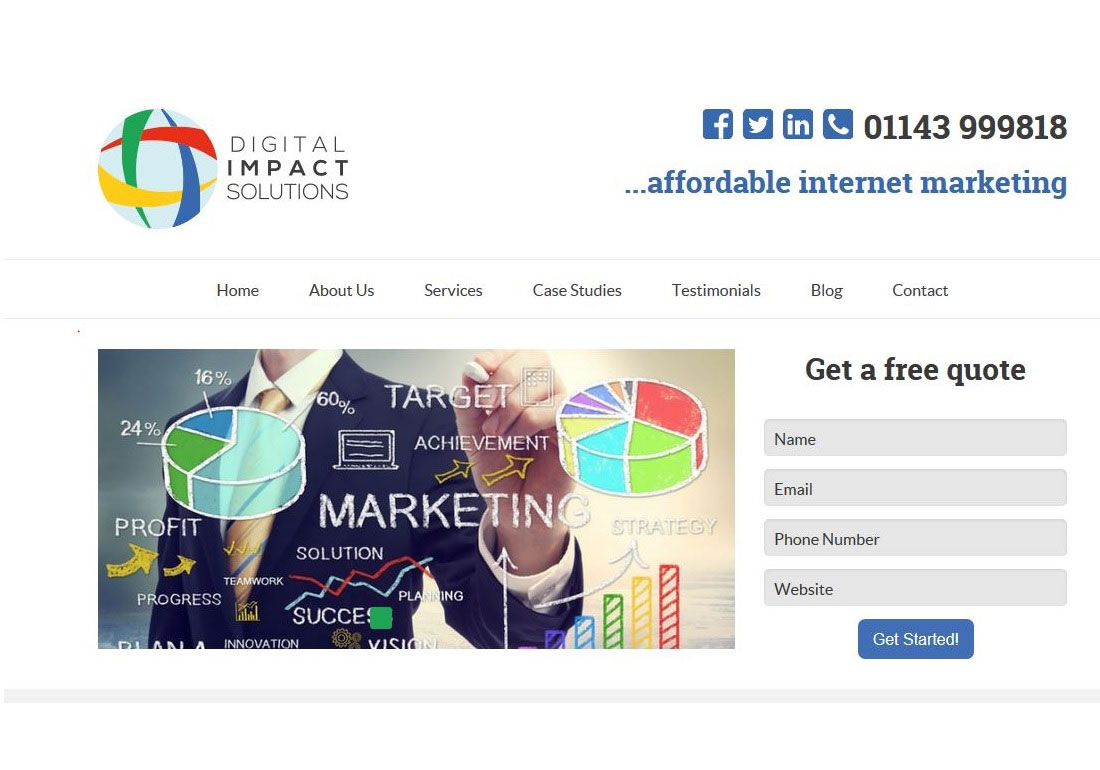The image depicts a screenshot of a horizontal, rectangular desktop webpage featuring a sophisticated and professional design. In the upper left-hand corner, there is an icon, a circle crafted from different colored, elongated triangles intricately woven to form a square basket weave pattern. Adjacent to this icon, the text "Digital Impact Solutions" is prominently displayed.

Positioned in the upper right-hand corner are various social media icons, along with a phone icon and the contact number 011-439-99818. Alongside this, the phrase "Affordable Internet Marketing" is clearly visible.

Below this section lies a navigation menu bar with the options: Home, About Us, Services, Case Studies, Testimonials, Blog, and Contact, providing seamless website navigation.

Beneath the toolbar, there is a stock photo featuring the torso of an individual dressed in a suit coat, tie, and dress shirt. The person appears to be holding a piece of chalk, extending it toward the viewer. Superimposed on this image is text, stylized to look as though it has been scribbled in chalk, accompanied by a pie chart detailed with the terms: profit, marketing, progress, teamwork, success, target, achievement, strategy, planning, vision, and innovation. Additionally, there is an illustration of a bar graph.

To the right of this visual content, a form invites users to "Get a Free Quote," requesting their name, email, phone number, and website details.